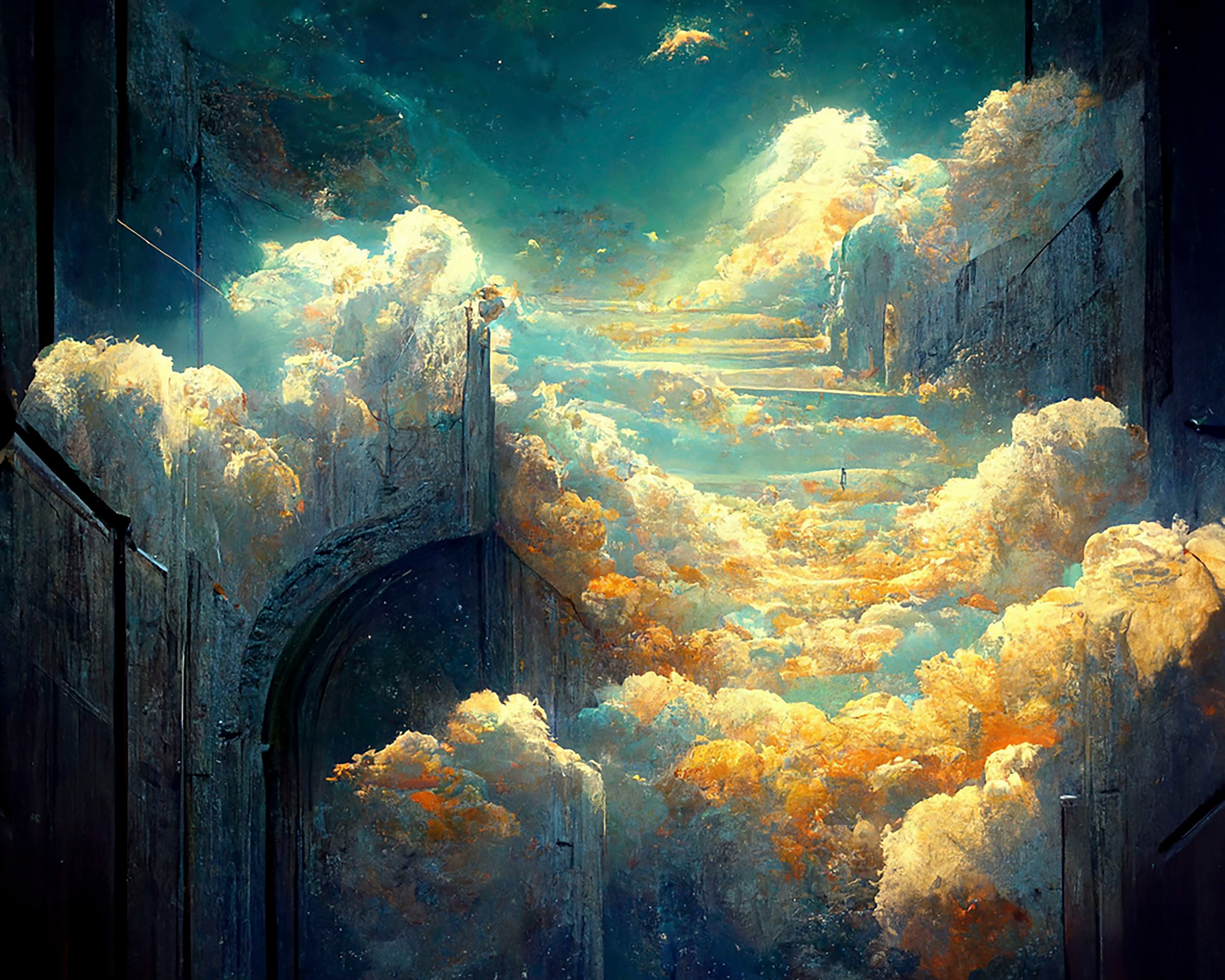This abstract and textured painting predominantly features shades of blue, with darker hues on the sides transitioning to lighter, more colorful tones towards the center. It creates a close-up view of what appears to be a mystical or surreal city in the sky. In the foreground, vibrant orange and yellow clouds, tinged with blue, seem to spill over the edges of what might be stone walls or buildings. These clouds are intermixed with cream and white highlights, suggesting an ethereal stairway ascending into a rich teal sky, evoking a "stairway to heaven" motif. Gold accents dot the sky, enhancing the celestial atmosphere. On the lower left, a darker navy archway anchors the scene, which is encircled by what resemble bushes or additional clouds. The painting merges into a nighttime sky with stars visible in the distance, further contributing to its dreamlike and abstract quality.